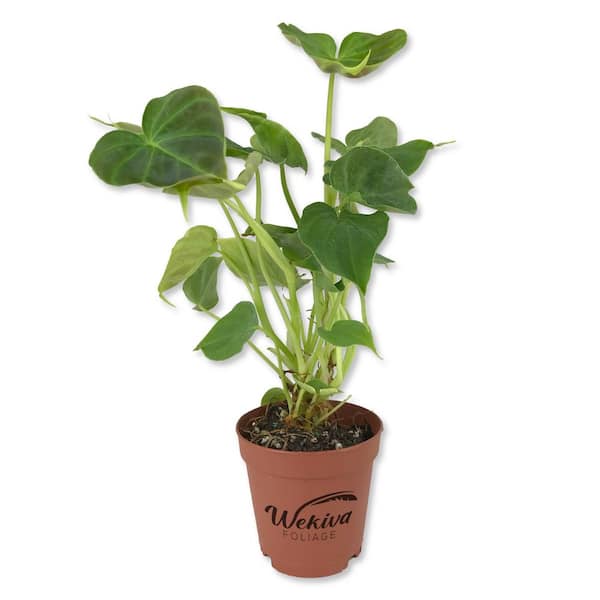The image features a tall philodendron plant with long, broad, dark green leaves and lighter green stems, emerging robustly from a pot. The plant is rooted in rich soil, housed within a brown planter. The planter bears the name "Wekiva" in bold black letters, with the letter W creatively designed to extend upward and resemble a leaf. Beneath "Wekiva," the word "foliage" is inscribed, emphasizing the botanical theme. The entire setup highlights the vibrant greenery and the elegant design of the planter, focused solely on the plant without any background distractions.